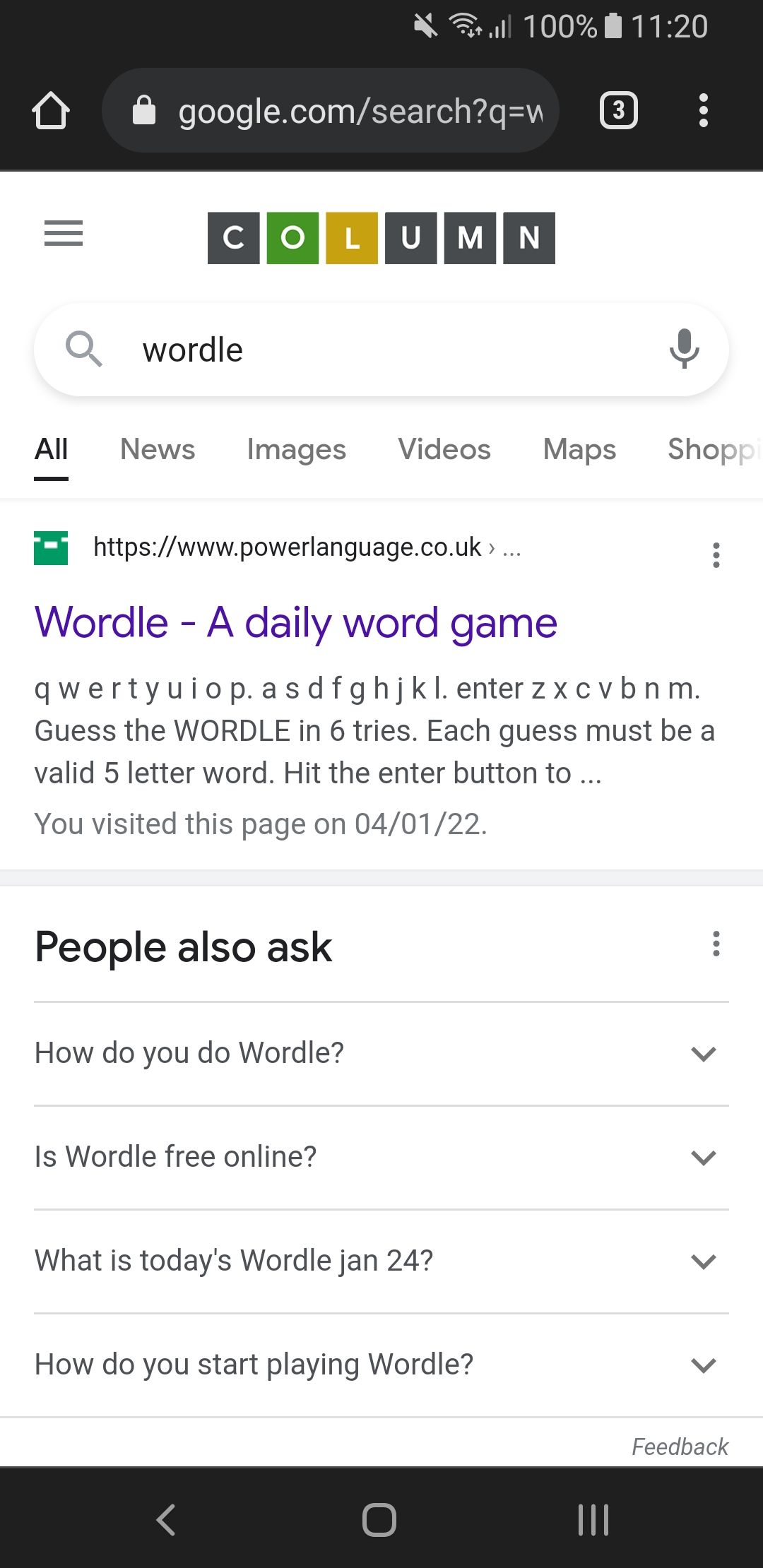The image is a portrait-mode screenshot of a smartphone displaying a Google search page. At the top, the status bar shows a battery life of 100% and the time, 11:20. Beneath this, the URL bar indicates the search inquiry is "google.com/search?q=Wordle". There are three open tabs visible, alongside a menu represented by three dots.

The next row presents the navigation options, with a three-line menu icon on the left, followed by the word "COLUMN." This row features the word game Wordle, where the letters "C-U-M-N" are on a black background, "O" is highlighted in green, and "L" is highlighted in yellow.

Directly underneath is the search bar where "Wordle" is typed, with an option for voice search available. Below the search bar are various Google search tabs: "All" (bold and underlined to indicate the current tab), "News," "Images," "Videos," "Maps," and "Shop."

The following result shows "Wordle - A daily word game" as a purple link, indicating it has been visited before, associated with the URL powerlanguage.co.uk. The game invites users to "Guess the Wordle in six tries. Each guess must be a valid five-letter word. Hit the enter button," with a note that the page was last visited on April 1, 2022.

Further down, a section labeled "People also ask" contains commons questions about Wordle, such as, "How do you do Wordle?", "Is Wordle free online?", "What is today's Wordle January 21, 2024?", and "How do you start playing Wordle?"